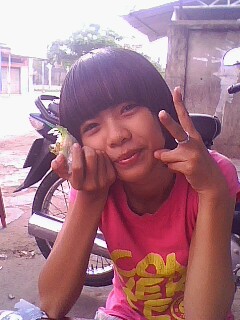This color photograph in portrait orientation features an Asian child with a bowl cut haircut and bangs, posing cheerfully for the camera. She is seated at a brown wooden table, smiling with her head tilted slightly to the left, her gaze directed up towards the viewer. The child is wearing a short-sleeved pink graphic t-shirt with yellow lettering, though the text is not readable due to the wrinkles and her seated position. Her elbows rest on the table; her left hand is raised, displaying a peace sign with her index and middle fingers, adorned with a silver ring on the middle finger. Her right hand, propped against her cheek, holds a partially eaten wrap with visible lettuce. In the background, partially obscured by her body, there is a scooter with black rubber tires, silver rims, and a black seat. Further behind is a flat-walled brown building with a straw roof, suggestive of a sunny day outdoors. Visible to the left is a portion of a tree and another white building. The setting and style of the photograph lend a sense of realism and vibrant everyday life.